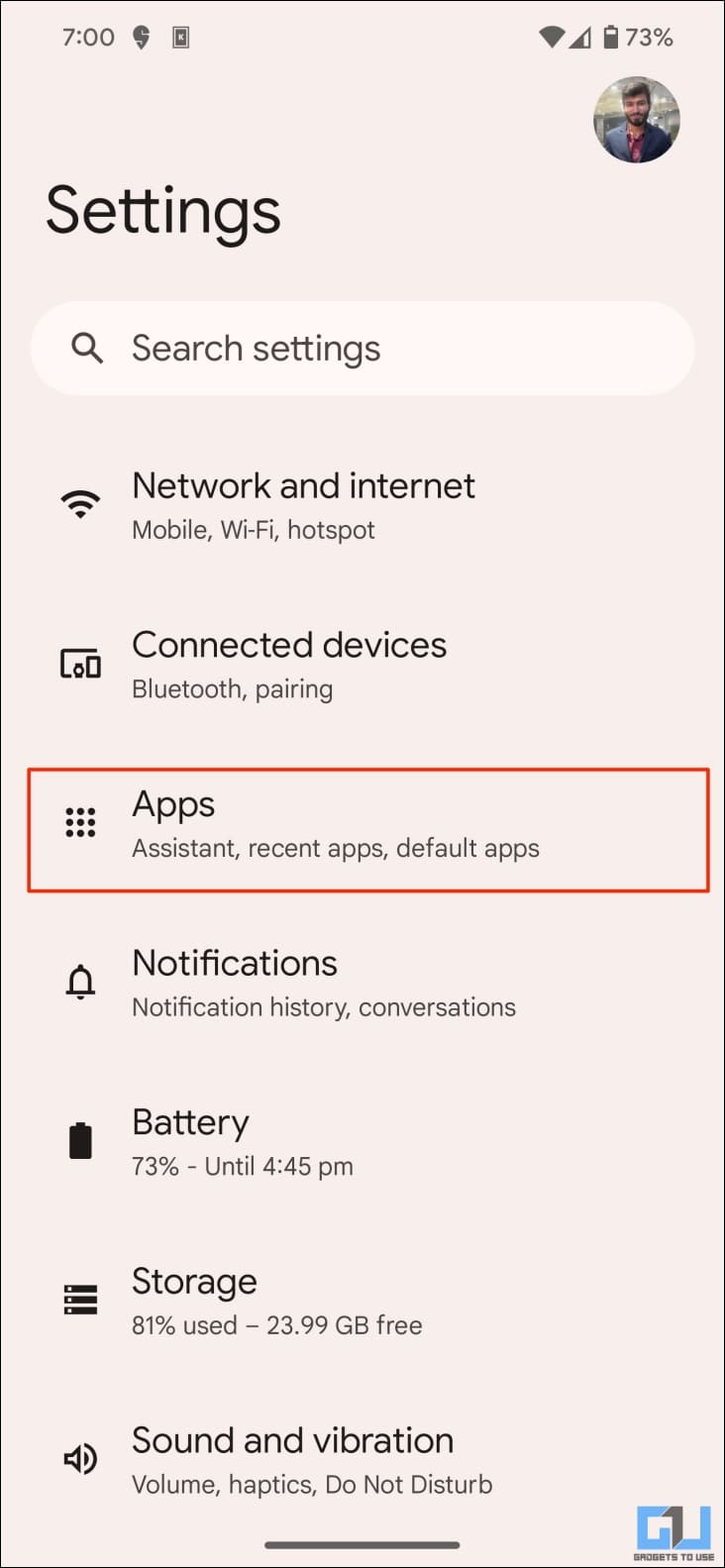This image is a screenshot taken from a cell phone, presented in a vertical rectangular format. The background of the interface is a soft, light pink. At the top of the screen, the status bar displays essential information: the time is set to 7:00, which is visible in the upper left corner. On the upper right, the Wi-Fi symbol indicates connectivity, and next to it, the battery icon shows a charge level of 73%. Directly beneath the battery icon, there is a small circular profile picture of a young man. He appears to be in his early twenties, with dark hair and a neatly groomed dark beard. The man, who is Caucasian, is smiling warmly at the camera and is dressed in a blue sports jacket.

Further down the screen, on the left side, large bold black text reads "Settings." Below this, a search bar labeled "Search Settings" is outlined by a light-colored oval, making it stand out. The settings menu lists various options: "Network & Internet," "Connected Devices," "Apps," "Notifications," "Battery," "Storage," "Sound," and "Vibration." The option "Apps" is notable as it is highlighted with a prominent red rectangle, indicating it has been selected. Within this selection, sub-options including "Assistant," "Recent Apps," and "Default Apps" are displayed.

In the bottom right corner of the screenshot, there is an unclear symbol that appears blue and black. The text near this symbol is difficult to decipher, but it seems to read something like "BroBets to Use."